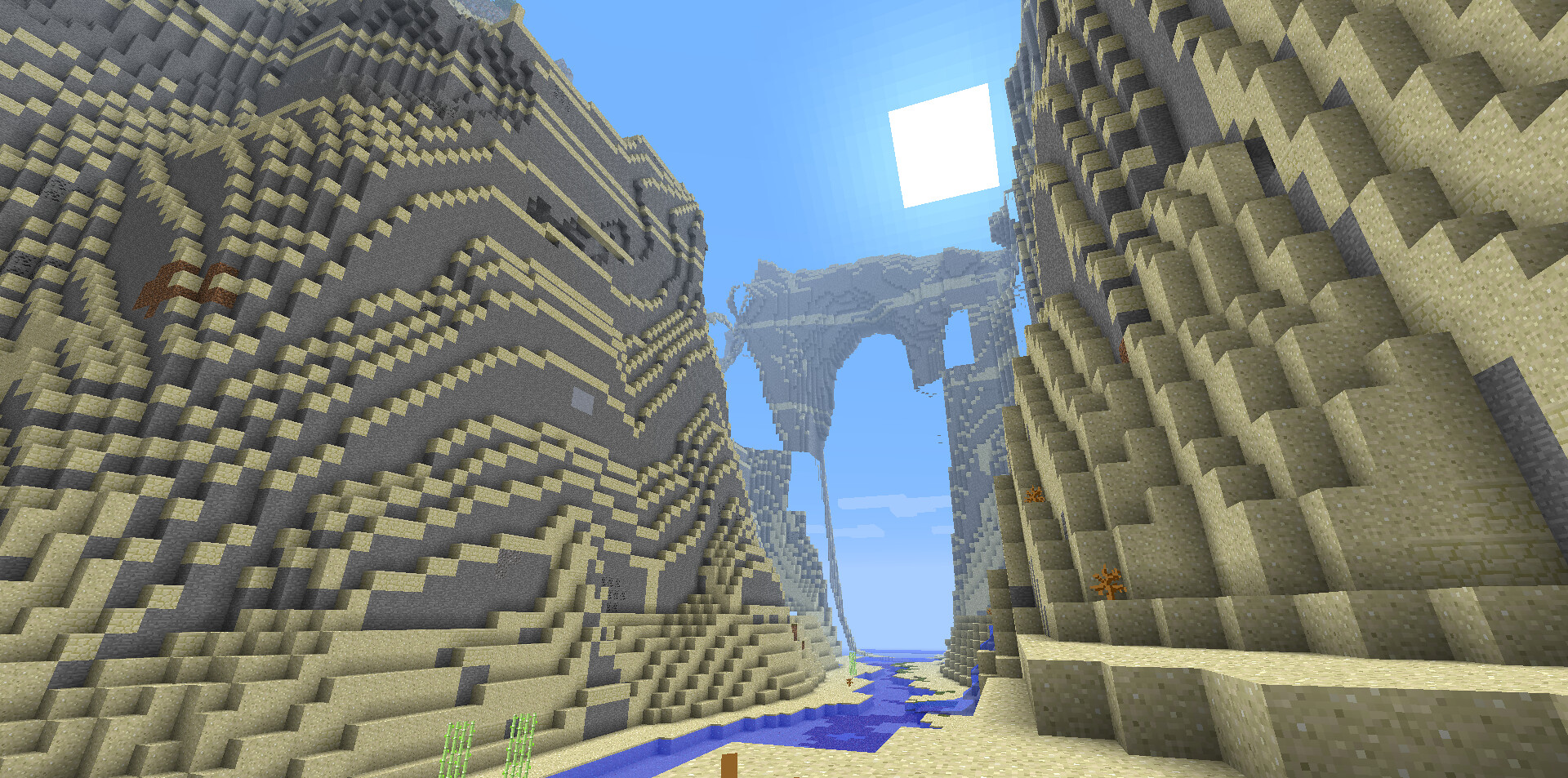The image depicts a computer-generated or video game scene characterized by a distinctly blocky, pixelated aesthetic reminiscent of Minecraft. It features two towering, white structures on either side that resemble monumental sandstone cliffs or mountains. These structures extend from corner to corner and are composed of various blocks, creating a stepped and squared appearance with a mix of light brown and dark brown hues. In the foreground, there's an orange-red creature, perhaps resembling a piece of coral, perched on some of the steps. Situated between these massive cliffs is a bluish river or stream, featuring gradations of dark and light blue, flowing through the scene. The background reveals a tall, arc-shaped structure with the river meandering through it, set against a blue sky. High above this arch is a prominent square-shaped white light, possibly representing the sun. Overall, the picture combines elements of abstract art and detailed, artificial landscapes within a rectangular frame.